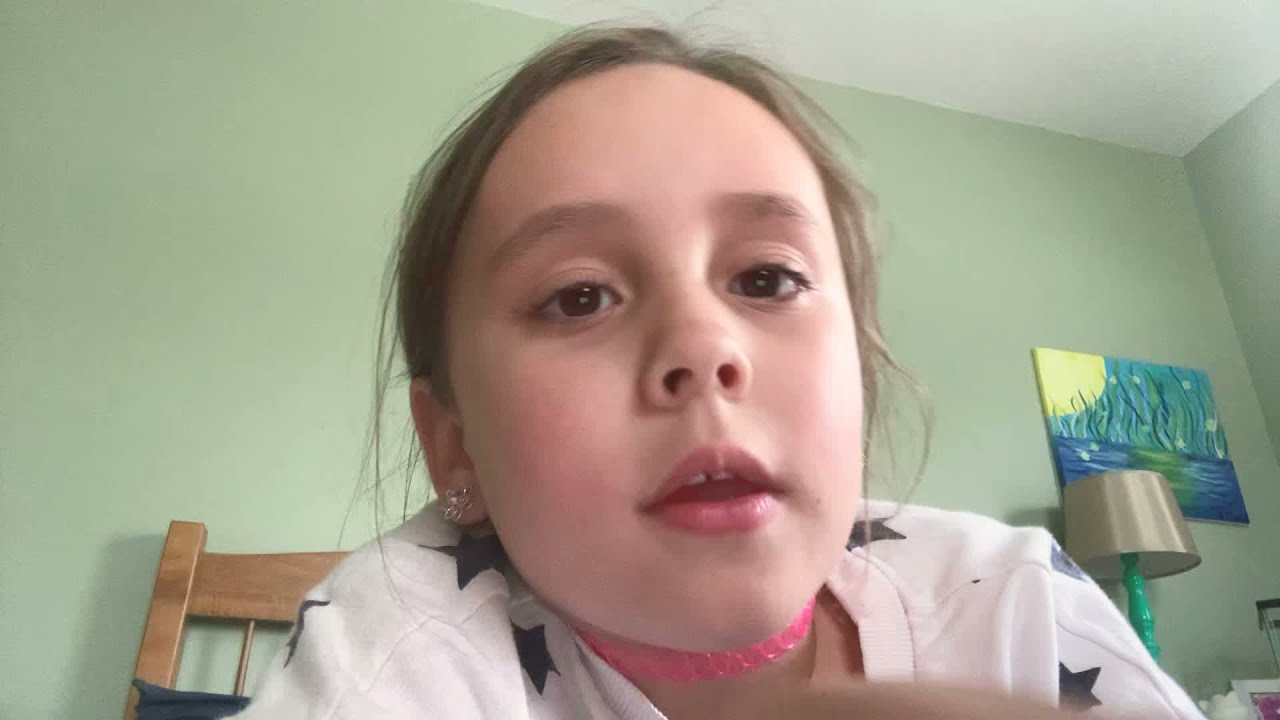In this detailed image, a young girl, approximately eight or nine years old, is positioned centrally, staring into what appears to be a computer or phone camera. She is up close to the camera, revealing her fair skin and hair pulled back with a few loose tendrils. She wears a white shirt adorned with black stars and a bright pink choker necklace, accompanied by diamond earrings. Her mouth is slightly open, adding a candid feel to the snapshot.

The setting is a room with light green walls and a ceiling in a much lighter shade of green. On the bottom left of the image, a corner of a wooden bed or chair is visible. To the bottom right, there is a painting depicting a body of water with the sun, resembling a piece potentially inspired by Vincent van Gogh. Underneath the painting stands a green lamp with a silver lampshade. The overall impression suggests this is her bedroom, with the cozy arrangement and personal items enhancing the intimate atmosphere of the scene.